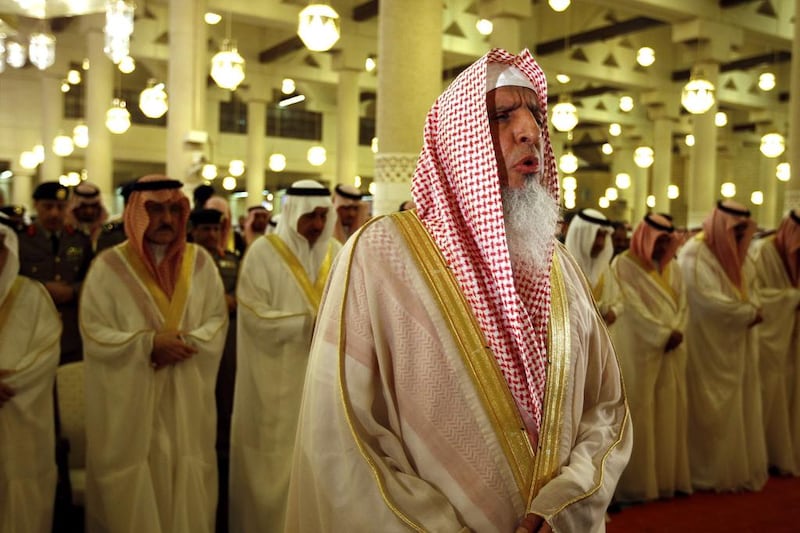This is a color photograph taken indoors, depicting a group of Arab men, likely from Saudi Arabia or a surrounding region, dressed in traditional attire. The men are lined up in columns, facing towards the right, and appear to be engaged in prayer. They are all wearing white robes (thobes) and head coverings, some purely white and others with the distinctive red and white checkered pattern known as a ghutra or shemagh. In the foreground, there is a distinguished older man with a white beard, also dressed in a white robe with a red and white headdress, who seems to be the leader of the group. Behind them, a few individuals in suits can be seen, possibly military advisors or personnel, indicating a more formal or official setting. The room is ornate, with elaborate hanging light fixtures and white pillars, reflecting a lavish and well-decorated interior. The overall scene captures a solemn and reverent moment in a grand and sophisticated environment, with a clear cultural and regional significance evident from the attire and setting.